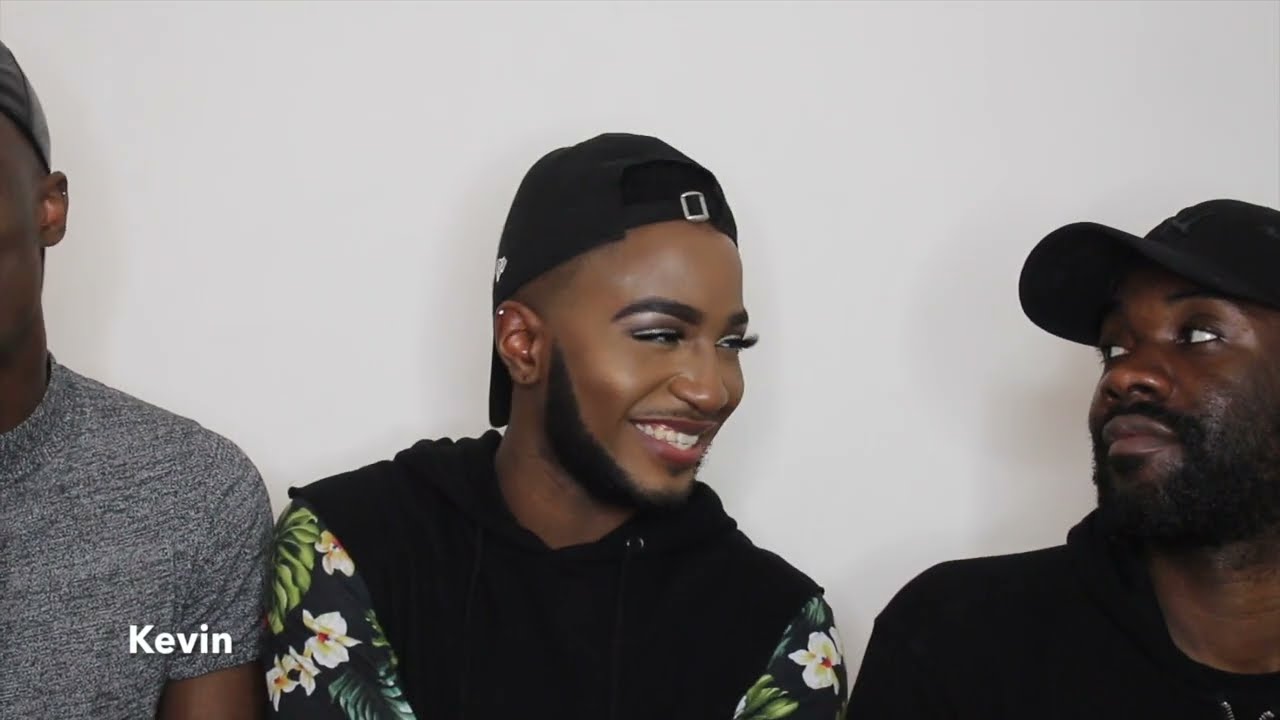In the image, three Black individuals are seated closely together, looking intently towards the camera, all set against a light gray indoor background. On the left, a man in a backward black ball cap and a gray sweater props his hands under his chin, giving an impression of attentive listening. The person in the middle stands out with noticeable makeup – including painted eyebrows, false eyelashes, eye makeup, and lipstick. They also have a small mustache and beard. This individual is wearing a black hat with a silver buckle, a black vest-like hoodie over a black shirt adorned with white flowers and green leaves, and is holding a fist near their face as if engaging in conversation. On the right, another man, dressed in a black hoodie with a silver zipper and a backward hat, sits slightly leaned back with his head cocked to the side, appearing deeply engaged. Shadows on the wall behind them suggest the photograph was taken indoors, capturing a moment of focused attention in a representational style.